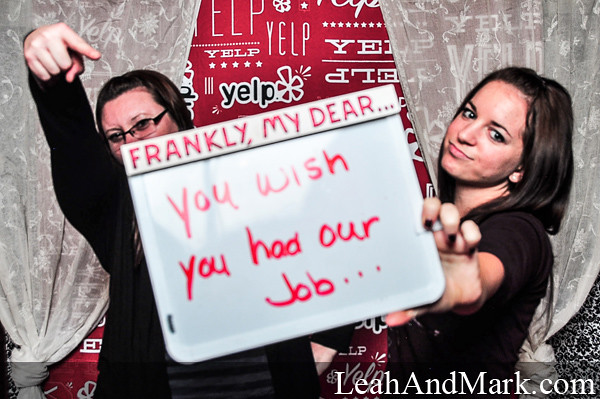The photograph, in horizontal orientation, features two women posed in front of a red backdrop with various iterations of the Yelp logo. The woman on the left, an older white woman with black-rimmed glasses and a black top, has her arm raised and is pointing towards a small white sign with red lettering. The woman on the right, a younger white woman with long black hair wearing a black top, is holding the sign, which reads, "Frankly, my dear, you wish you had our job..." The sign is slightly tilted. Adding to the composition, sheer white lace curtains adorn both sides of the background, partially covering the Yelp logos. At the bottom right corner of the image, the website leahandmark.com is visibly imprinted as a watermark. The overall scene suggests a promotional or recruitment photo for Yelp.